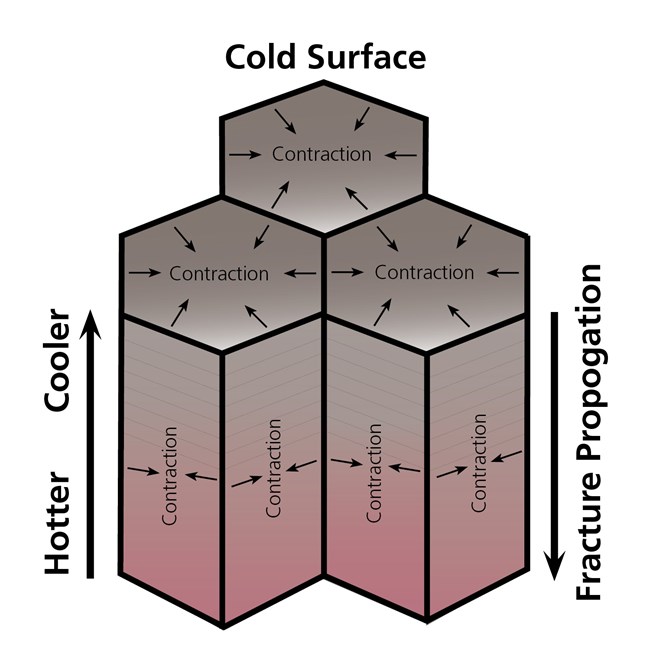The diagram features a detailed schematic illustrating temperature and fracture propagation. On the far left, there is a vertical gradient labeled "hotter" at the bottom and "cooler" at the top, with a black arrow pointing upward to indicate decreasing temperature. At the top of the diagram, there is a label that reads "cold surface" in black text. To the right, a vertical arrow labeled "fracture propagation" points downward, symbolizing decreasing fracture propagation.

In the center of the diagram, there is a complex structure composed of multiple geometric shapes. The upper section comprises a gray and red hexagon with arrows pointing inward to the center, labeled "contraction" seven times. Below this, there are associated shapes, including three interconnected hexagons and four parallelograms, all of which also have arrows converging towards their centers and are labeled "contraction." The entire diagram is set against a white background, further emphasizing the structural and temperature-related annotations.